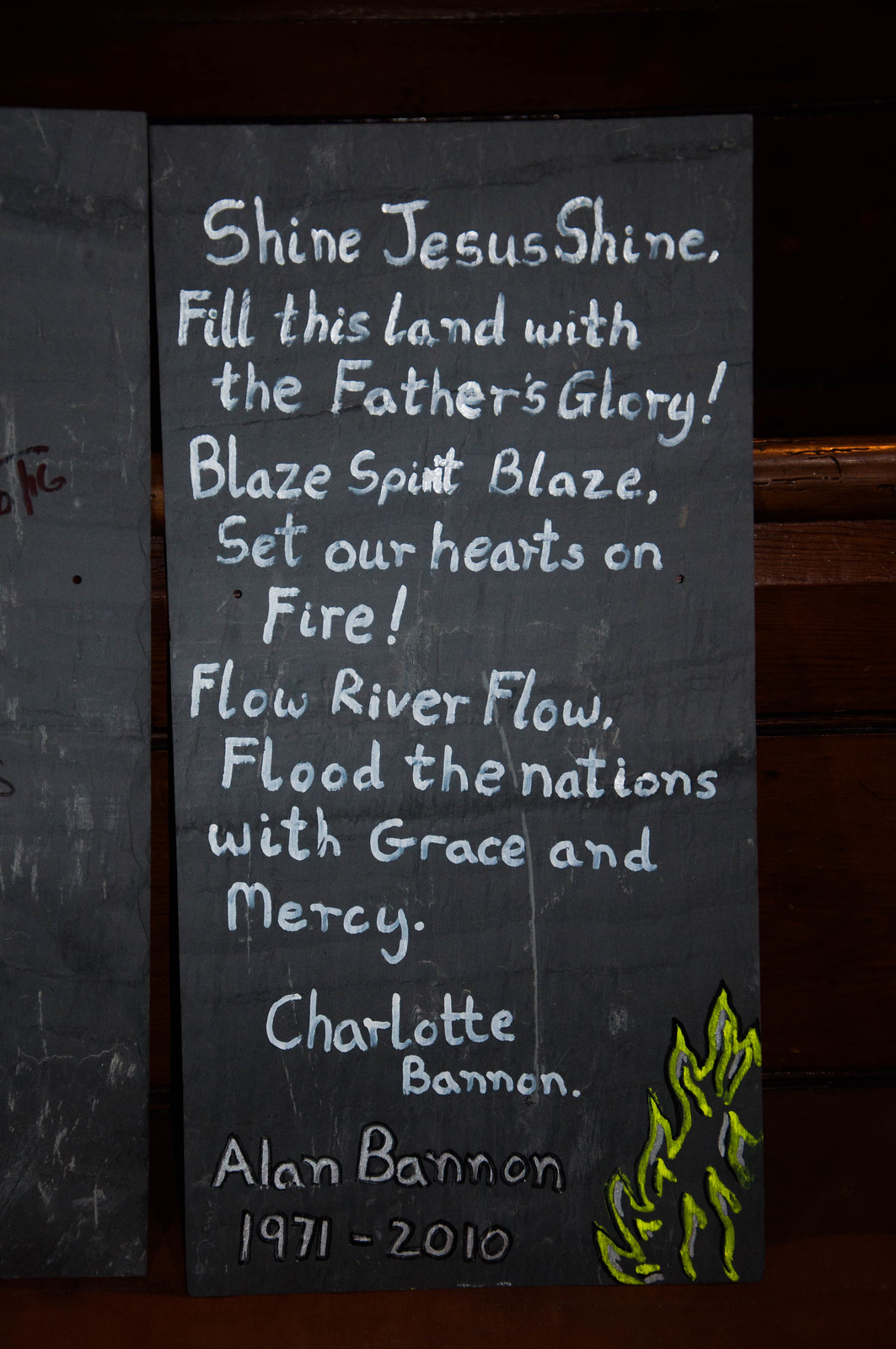The image depicts a blackboard with a poignant, vertically written text in white chalk: "Shine, Jesus, shine. Fill this land with the Father's glory. Blaze, spirit, blaze. Set our hearts on fire. Flow, river, flow. Flood the nations with grace and mercy." Attributed to Charlotte Bannon, the inscription serves as a heartfelt tribute. Below, in a lighter shade, the name "Alan Bannon, 1971 to 2010" appears, marking a commemorative note for a life lost too soon at the age of 39. Enhancing the memorial's visual impact, neon green chalk illustrates flames in the lower right corner, symbolizing the blazing spirit and enduring memory of Alan Bannon. The combination of text and illustration creates a deeply touching homage.